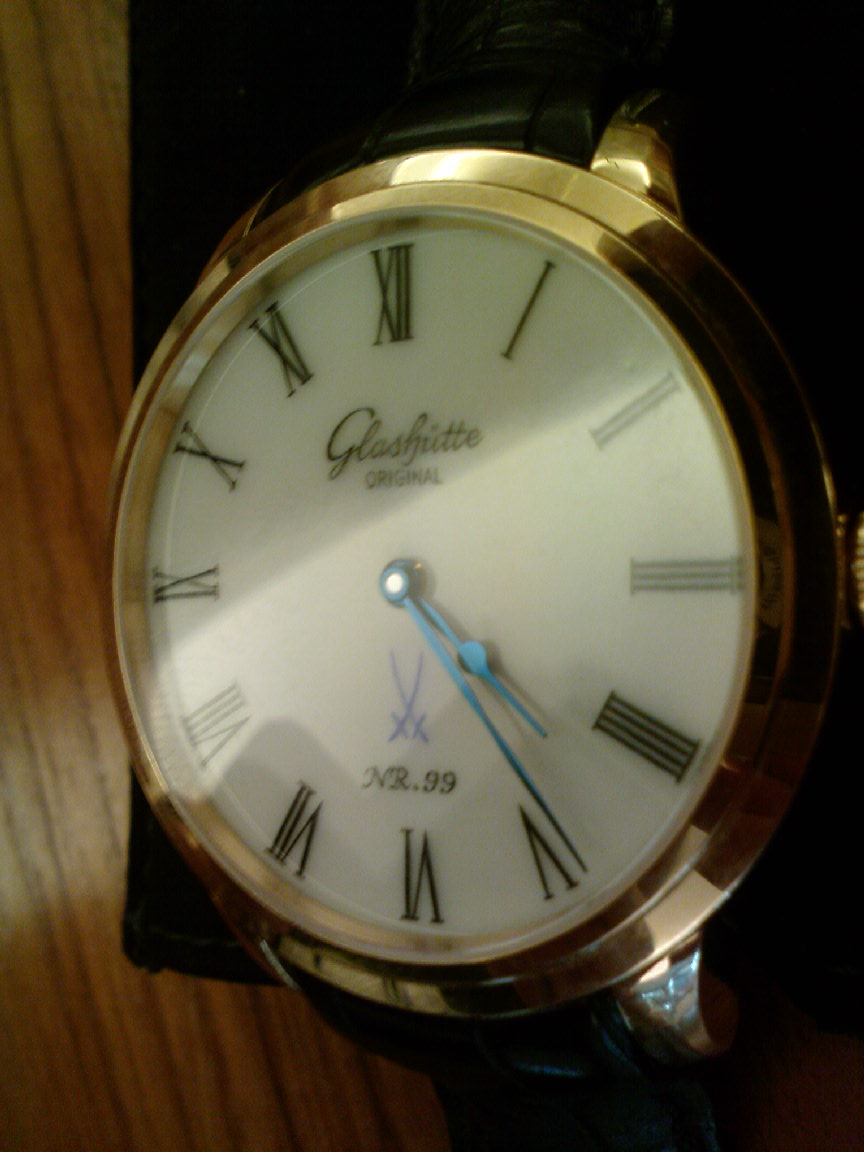The photograph is a close-up shot of a luxury wristwatch nestled in a black velvet-like fabric case. The background fabric provides a stark contrast against a visible wood surface with distinct wood grain patterns, suggesting a dark oak table. The watch features a gold-colored case with a black or dark leather strap, though only the edges of the strap are visible at the top and bottom of the frame due to the cropping.

The watch face is white with gold or bronze Roman numerals, and it is adorned with blue hour and minute hands, showing the time as 4:24. Notably, there is no second hand. Just below the 12 o'clock position, in cursive script, it reads "original Glashütte," albeit with the name slightly blurred and difficult to decipher. At the bottom of the dial, the inscription "NR.99" is clearly visible in black. A simple yet elegant crossed swords logo, composed of blue lines, is positioned just below the watch hands, balancing the sophistication with a touch of subtlety. This macro photograph captures the intricate details and luxurious elements of the timepiece, despite the slightly challenging readability of the brand name.